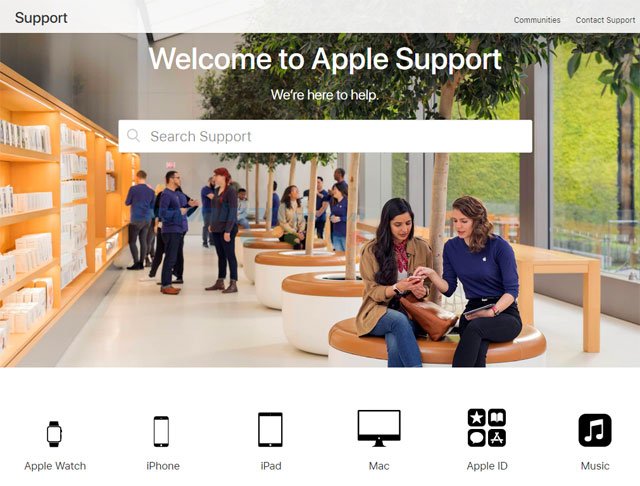The image features a welcome screen for Apple Support prominently in the center. At the top, the header contains "Support" in the upper left, and "Communities" and "Contact Support" in the upper right corners. Beneath the large text "Welcome to Apple Support," a subtitle reads "We're here to help," followed by a white search bar containing the placeholder text "Search Support" alongside a search icon.

The background showcases a modern space bathed in natural light streaming through large windows. Arranged in this room are planters with trees surrounded by seating areas, totaling six planters. To the left, a series of bookshelves adds structure to the scene.

Below the main greeting and search bar is a navigation row with options: "Apple Watch," "iPhone," "iPad," "Mac," "Apple ID," and "Music," spanning from left to right.

The color palette is a harmonious blend of gray, white, golden brown, cream, tan, blue, pink, green, silver, and black. These colors are not only present in the photograph but also reflected in the attire of the individuals within the space, contributing to a cohesive and inviting atmosphere.